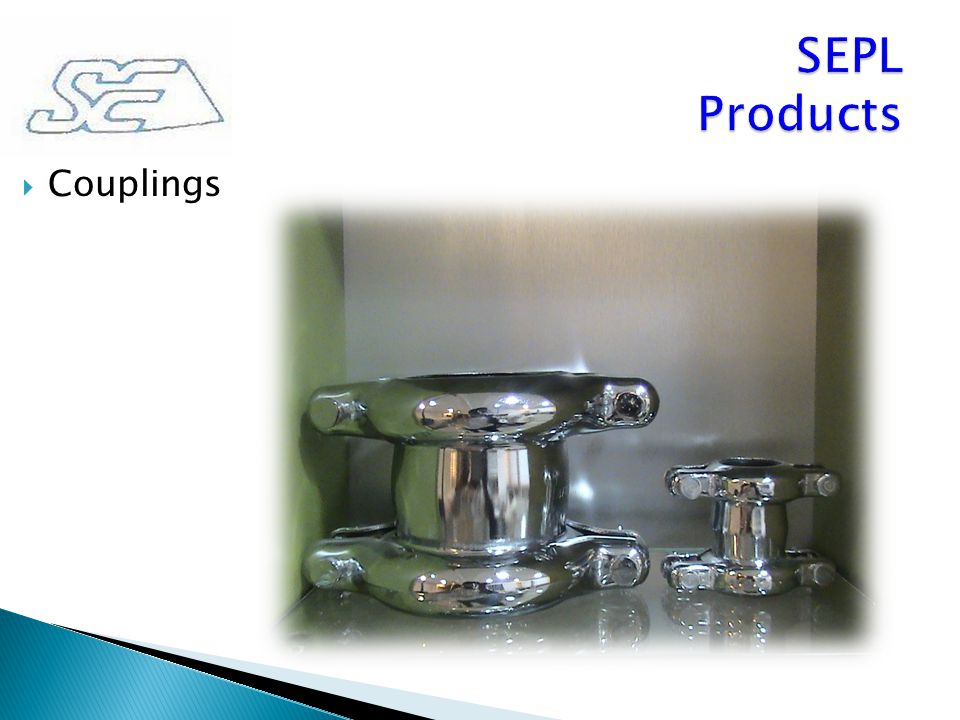This image appears to be a detailed catalog entry or advertisement for industrial couplings, potentially part of a PowerPoint presentation. In the center, there's a color photograph featuring two chromed, cylindrical metal fixtures, likely made of stainless steel, with reflective surfaces. These are positioned in a box that features green sides and a white back, which gradually fades into the white background of the slide.

The top left corner of the slide displays a logo composed of the letters "SC" connected by a line forming a rightward-pointing blue triangle, accompanied by a word in black text that reads "Couplings." The top right has the text "SEPL Products" written in blue, with "SEPL" fully capitalized and "Products" capitalized at the beginning. 

In the bottom left corner, there are several overlapping geometric shapes, including a blue, black, and lighter blue or grey triangle making up part of the slide's border. These elements collectively contribute to the professional and visually structured layout of the presentation slide.